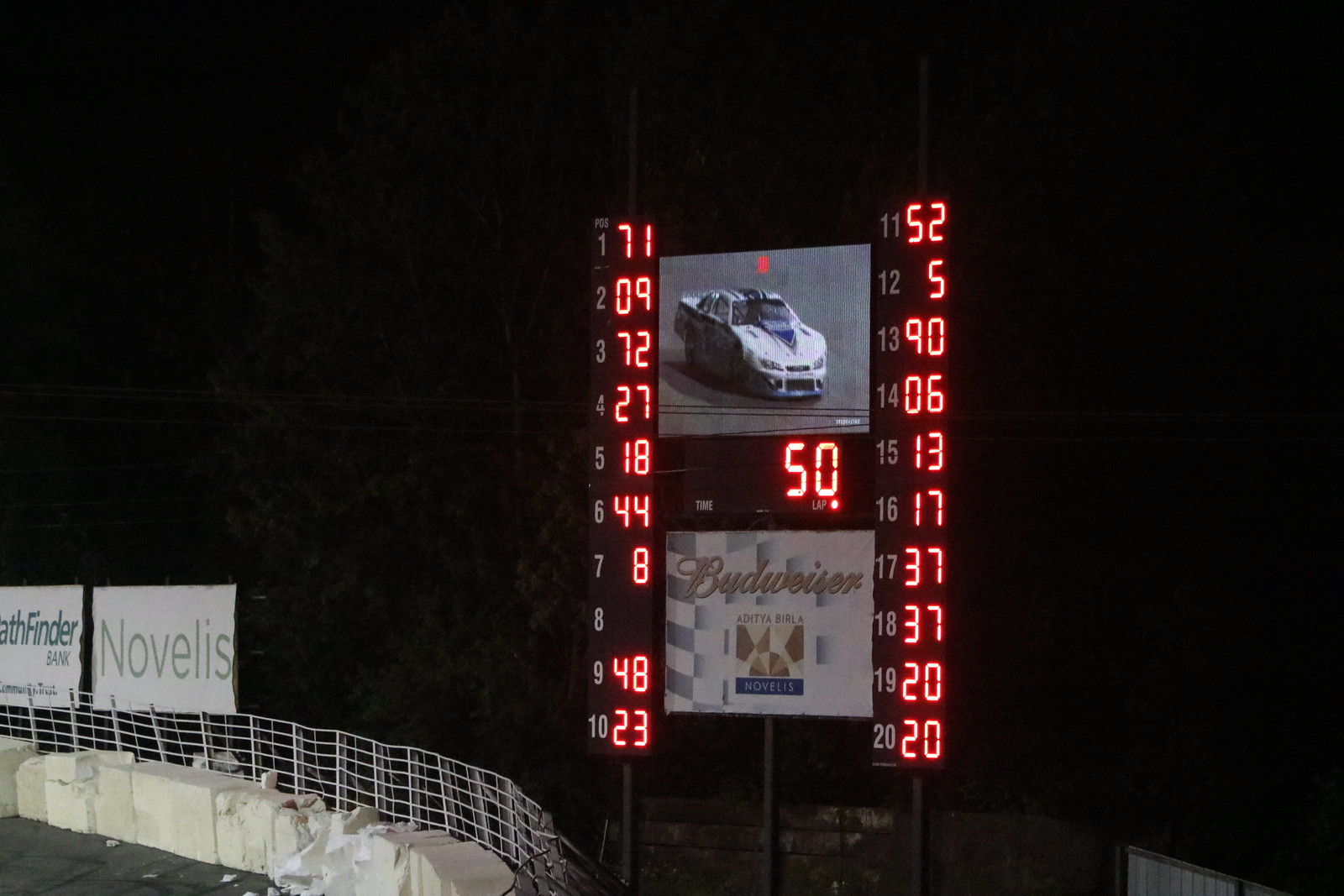This image, taken on a dark night at a small racetrack, showcases a detailed scene with various notable elements. Dominating the scene is a tower-like scoreboard structure, elevated by three black metal pillars, positioned prominently against the black night sky. The scoreboard features a central digital readout displaying the number '50' in red digital font. Directly above this readout is a square video board depicting a race car, likely white and blue in color. Beneath the digital readout, an advertisement for Budweiser, marked by white with gold lettering, is visible.

On either side of the central digital readout are vertical columns showcasing numbers that indicate the positions of race cars, ranging from 1 to 20. The numbers are arranged non-sequentially, with duplicates like '37' and '20' appearing, and range from as low as '5' to as high as '72'.

In the lower left corner of the image, part of the racetrack is visible. This includes a curved section of the track bordered by a white retaining wall, which shows signs of past collisions, and a wired net fence above it. Additional features include tarmac, a few hay bales for cushioning, and advertising boards. The advertisements, situated just above the retaining wall and on the fence, promote ‘Novalis’ and a partially obscured name that includes the word 'finder.'